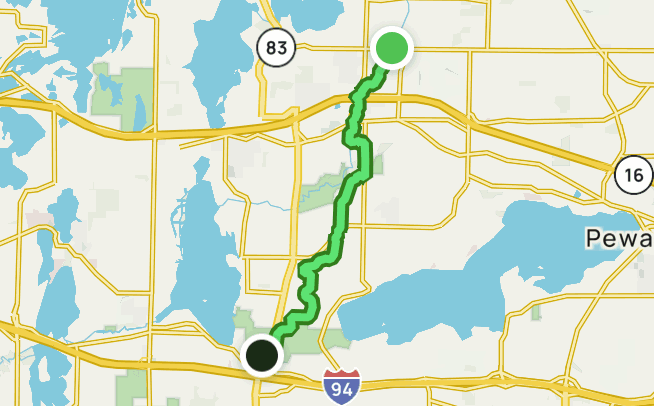The image is a detailed map featuring a light green circle with a white outline at the top and a dark green circle with a white outline at the bottom, connected by a light green pathway with a dark green border. The map includes various markings: a white circle with a black border indicating the number 16 on the right side, and another circle with the number 83 at the top left. There's also a blue highway shield with a red top labeled 94. The land areas are depicted in beige or light yellow, while the bodies of water are light blue. Yellow roads with darker yellow contours spread across the map. A partially visible name, beginning with the letters "PEWA," hints at the town or city depicted. The map appears to be a digital rendering, likely sourced from the internet.